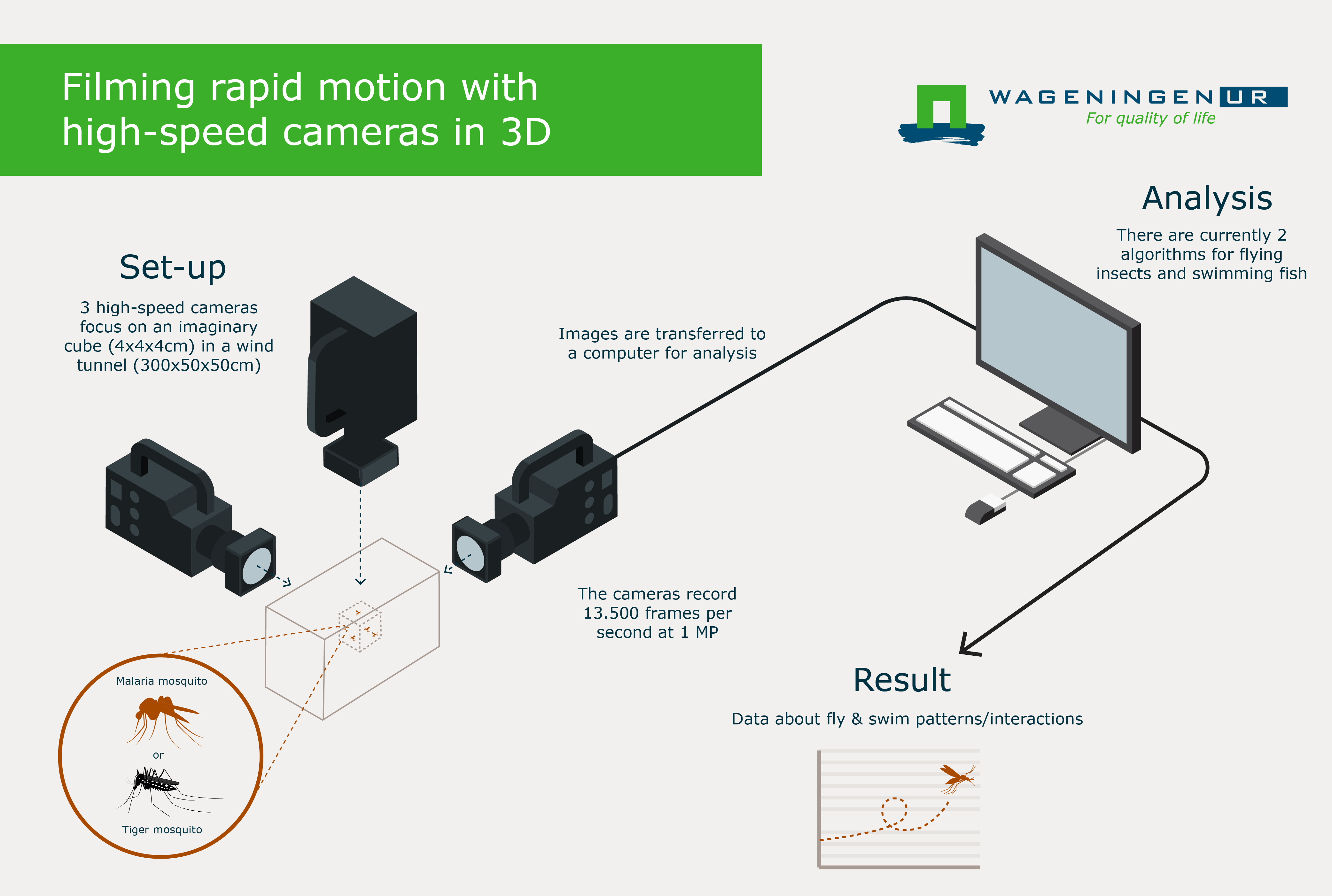Here is the cleaned-up and detailed caption:

---

This image, resembling a slide from a PowerPoint presentation, visually explains the process of capturing high-speed, rapid-motion photographs in 3D using specialized cameras. The background of the image is white, with several annotated diagrams detailing the procedure.

At the top left, a green rectangle contains white text stating "Filming Rapid Motion with High-Speed Cameras in 3D." Adjacent to this, on the top right, is a green and blue company logo for Wagening UR, featuring a structure resembling goalposts—a straight line with two horizontal lines descending at 90 degrees in green, with a blue line at the bottom. Below the logo, the tagline "For Quality of Life" is displayed.

The central illustration shows three high-speed cameras positioned at different angles, all focusing on a pair of mosquitoes enclosed within a box. One of these cameras is connected to a monitor, labeled "Setup." Annotations explain the setup: "Three high-speed cameras focus on an imaginary cube in a wind tunnel. Images are transferred to a computer for analysis. The cameras record at 13,500 frames per second with a resolution of one megapixel."

An arrow pointing from the cameras to the word "Result" highlights the subsequent stage—data analysis. This section notes: "Data about fly and swim patterns interactions," and shows an image of the mosquito movements captured by the high-speed cameras displayed on a computer screen.

Behind the monitor, labeled "Analysis," is further clarification: "There are currently two algorithms for flying insects and swimming fish."

Overall, the image effectively communicates how high-speed cameras are used to create detailed 3D visual records of mosquito movements, with the process being meticulously documented and annotated for clarity.